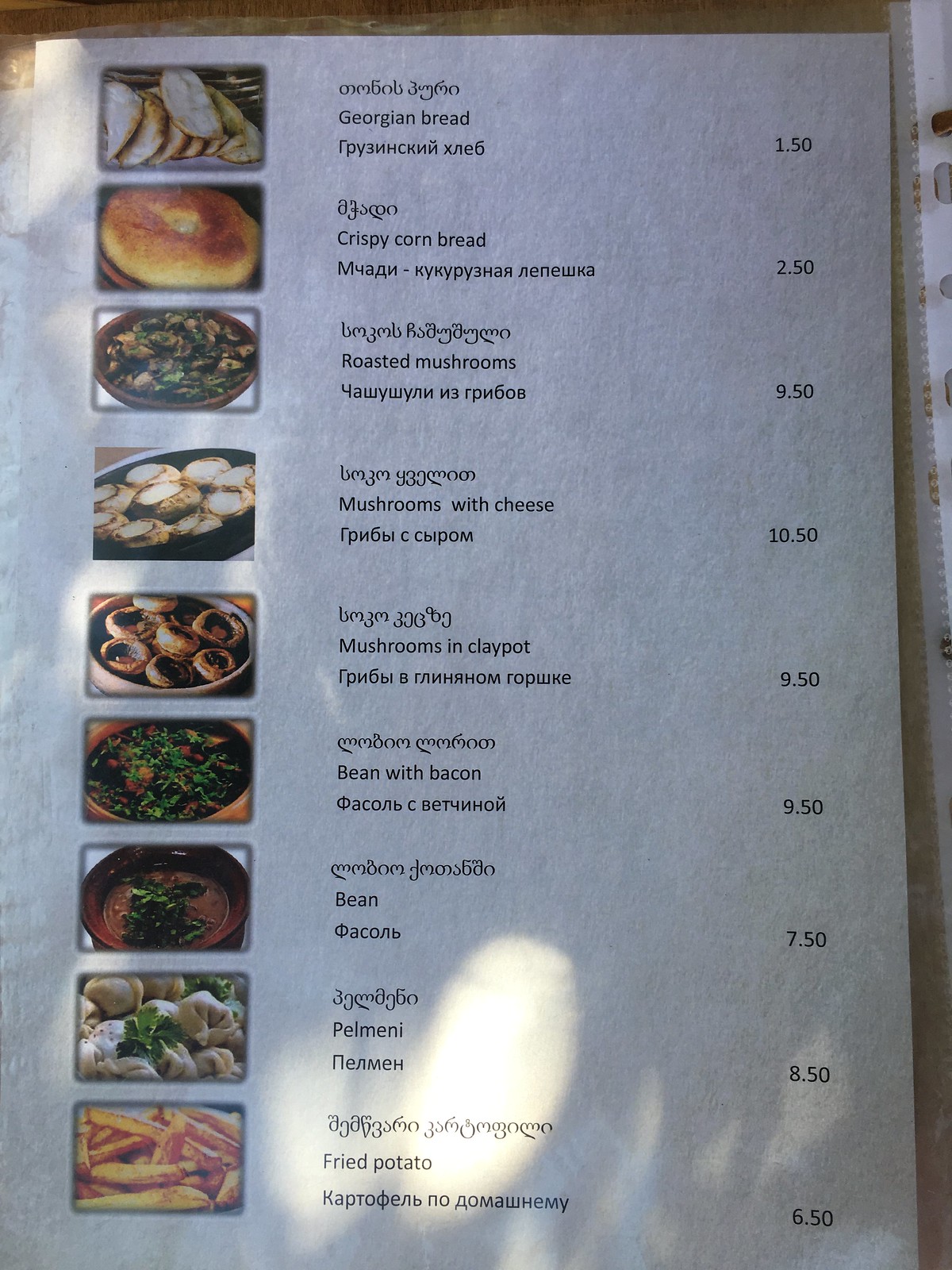The image is a tall, rectangular photograph of a multilingual restaurant menu propped up against an unseen surface, likely a table, based on faint edges visible at the bottom. The menu details various dishes, each listed in three different languages: Georgian at the top, English in the middle, and Russian at the bottom. Prominent dishes include "Georgian bread," mushrooms with cheese, beans with bacon, calamari, fried potatoes, roasted mushrooms, and crispy cornbread. Each dish is accompanied by a corresponding image and price, which range from 1.50 to 10.50, though the currency is unspecified. Reflections of sunlight, particularly visible in the lower section and the upper left corner, suggest the menu is either photographed outdoors or near a window.